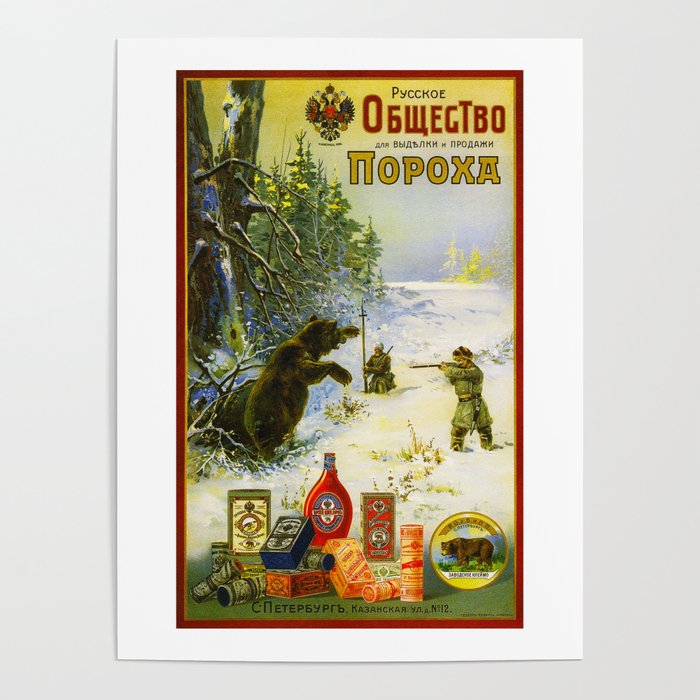This detailed Russian print advertisement features a dramatic scene set against a wintry landscape. Encased within a white border and a thin red inner border, the top of the image displays red and yellow Russian text along with a logo. The background showcases a blue sky tinged with yellow at the top, transitioning into snow-covered ground sprinkled with tall, green, and full trees. Dominating the scene is a striking confrontation between a brown bear standing on its hind legs and two Russian soldiers. One soldier, distinguished by a turban and a cross-like spear, also carries a gun over his shoulder, while the other soldier aims his rifle directly at the bear. In the foreground, various preserved and canned food products, including tins and a prominent red bottle, are carefully arranged. A distinctive cylindrical can featuring an image of a bear, similar to the one in the illustration, is also visible. The overall composition suggests an endorsement for fortified food items, possibly designed for survival in harsh conditions.